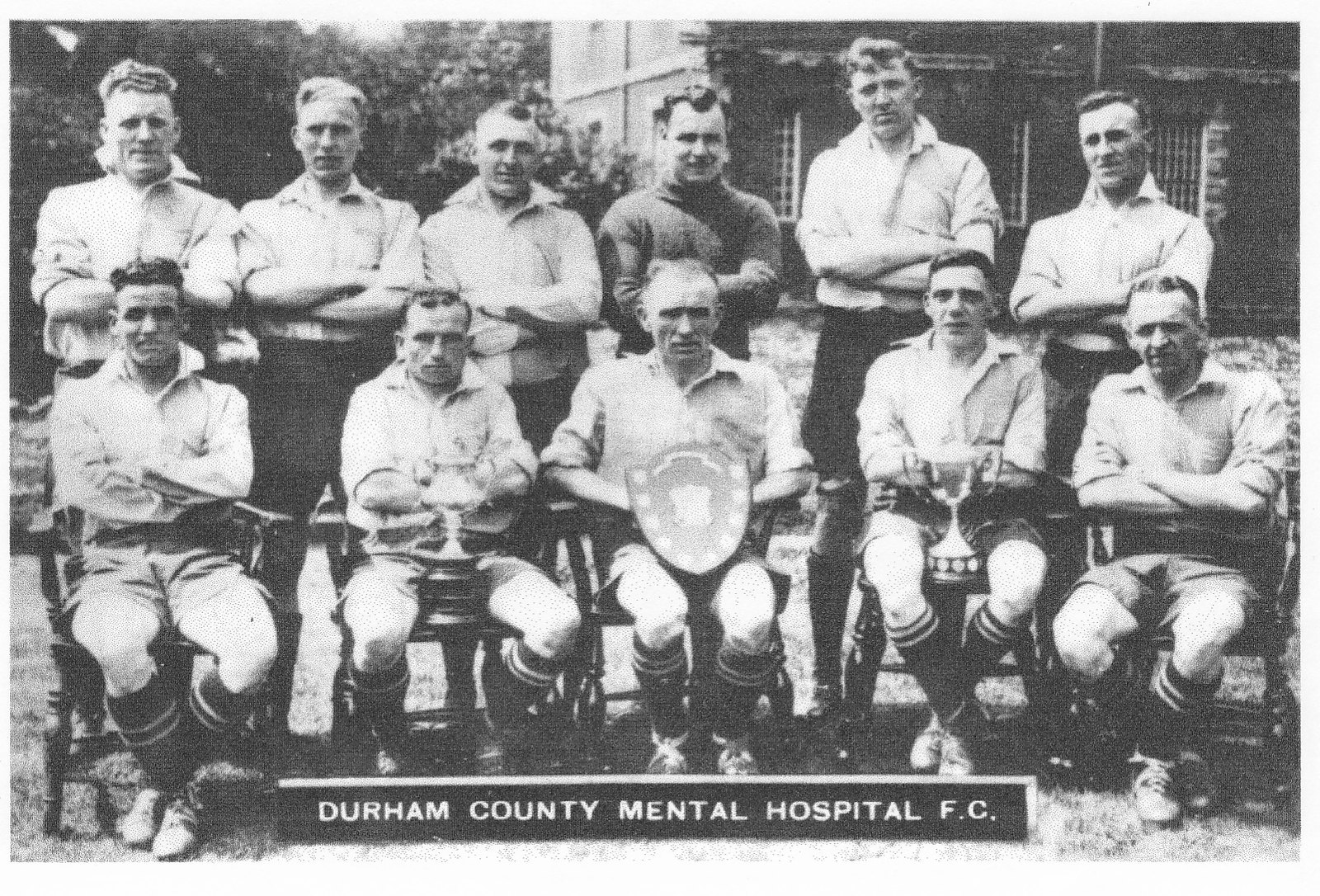This photograph is an older, black and white group shot of men, labeled "Durham County Mental Hospital FC" at the bottom. Comprising of a close-up of a photograph, the image includes eleven men, arranged in two rows: five seated in wooden chairs in the front and six standing behind them. The men, appearing to be aged between their 30s to 60s, display a formal demeanor, with most of them having their arms crossed. Noteworthy details include one man in the center of the front row who is holding a shield or emblem, while two other men in the front hold trophies in their laps, suggesting they were recipients of some awards. The backdrop features the top of some trees in the upper left corner and part of a building with visible rectangular windows in the upper right corner, partially cut off by the frame. The ground is grassy where the men are positioned.